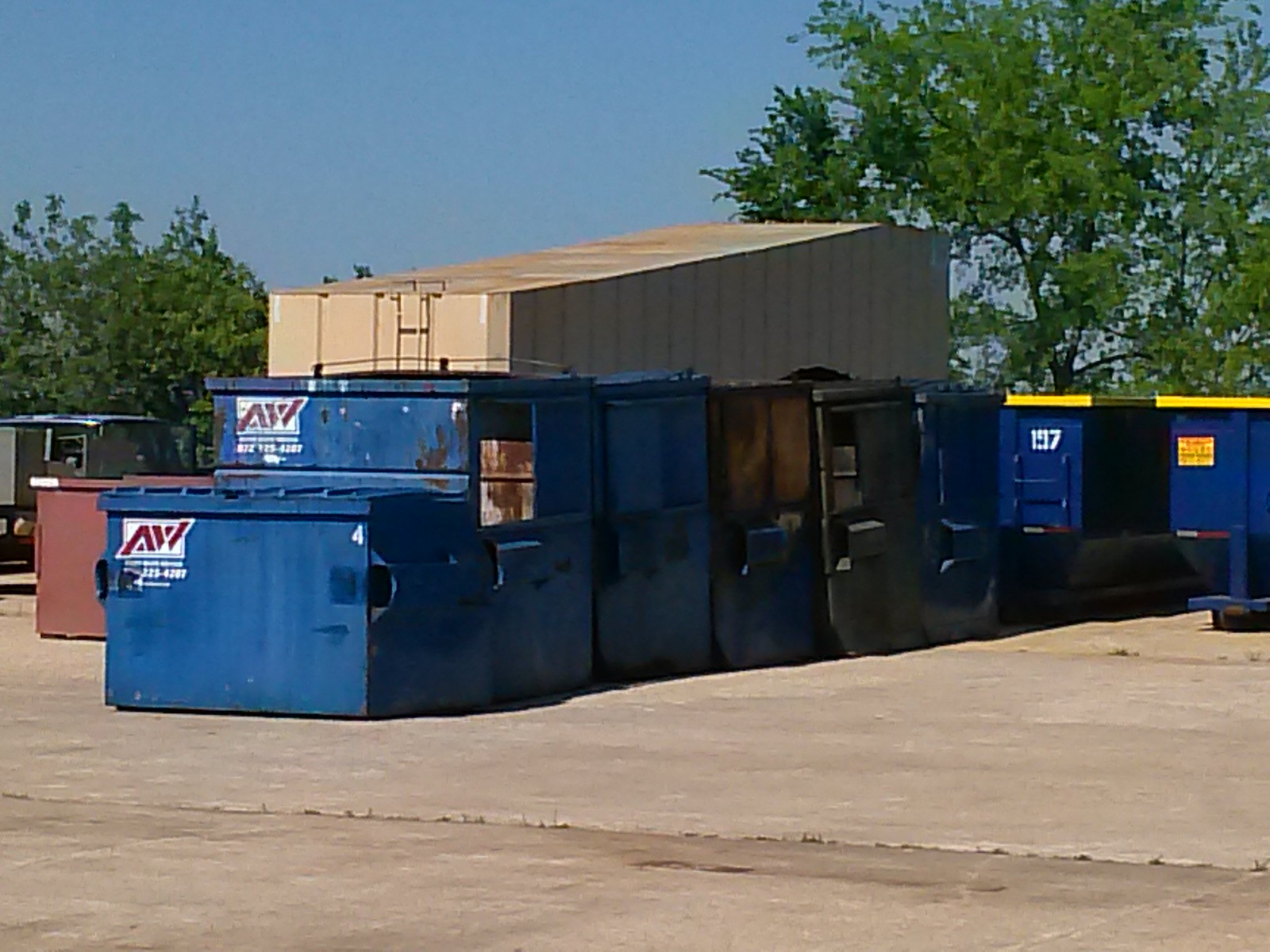In this outdoor daytime photograph taken under bright sunlight, a collection of six or seven blue dumpsters, some slightly differing in shades of royal blue and navy blue, are neatly arranged in a diagonal row from left to right. Each dumpster prominently displays a white rectangular logo with "AW" in white or red letters on the front. The foreground is paved in concrete, and the dumpsters are lit from the left side, casting shadows on their right. In the background, a large tan metal building with a slightly sloped roof stands behind the row of dumpsters. Additional features include a fully grown tree with leaves in the upper right corner, small bushes or shrubs on the left, a burgundy structure, and a green tractor trailer. The clear blue sky forms the backdrop, creating a stark contrast with the utilitarian scene below. Some of the dumpsters show signs of wear, such as scuffs, rusty marks, and dents. Notably, the dumpsters farther back in the row have yellow lids, while the others have blue or black lids, contributing to the varied blue hues against the gray paved lot.